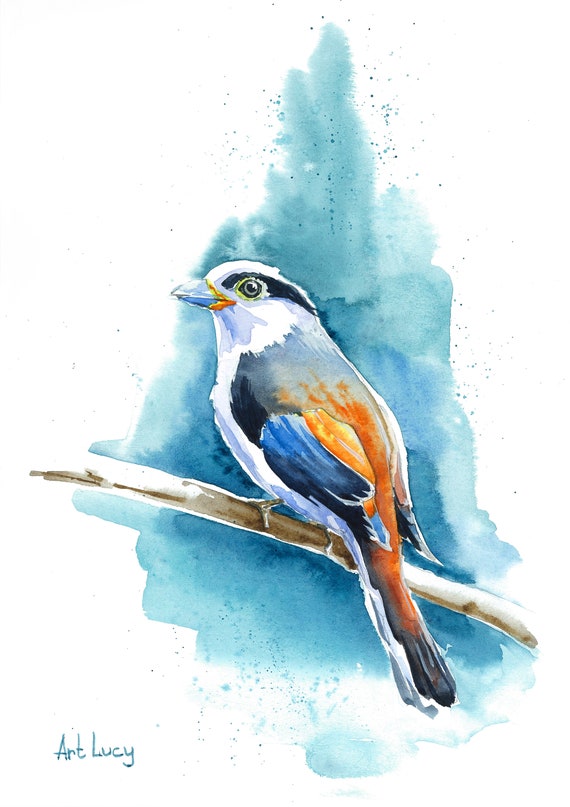The image showcases a detailed watercolor painting of a multicolored bird perched on a light brown branch. Identified by the signature "Art Lucie" in the lower left corner, the bird features a striking combination of colors. Its predominantly white head possesses blue splotches, while the beak is blue with a distinctive orange V-shaped marking where it meets the head. The bird’s eyes are black, encircled by yellow, and bordered by black streaks. Its wings display a vibrant mix of blue and orange, with the tail feathers transitioning from orange to a tipped black and white underside. The bird's belly is white, accented with orange splotches near the midsection and cyan towards the upper body just below the head. The branch it sits on has white splotches, contributing to a naturalistic texture. The background is primarily a gradient of cyan and lighter blue hues, forming a roughly triangular shape that frames the bird, adding depth and a splash of color to the white backdrop. The painting has a photorealistic quality, evoking the detailed style of classic Audubon illustrations.